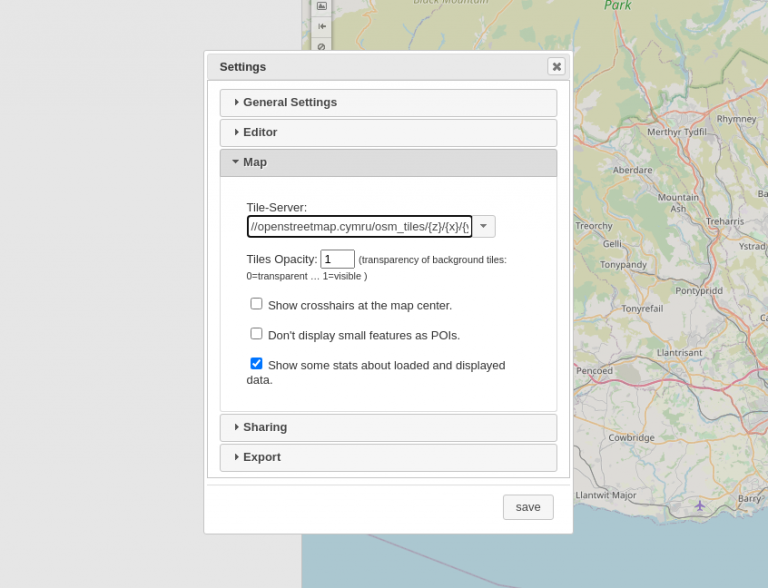The image is a screenshot of a digital map displayed on an app or website. The interface features a light gray background on the left side, while the right side prominently showcases a detailed map that includes both land and water areas. The land is depicted in a light mint green color, interspersed with darker green patches and beige regions, suggesting different types of land cover or uses. The water is represented in various shades of blue.

Multiple colored lines—red, blue, and orange—crisscross the map, possibly indicating routes, boundaries, or other significant features. Iconography on the map includes an airplane symbol situated at the bottom, hinting at an airport or flight-related information. Place names are also visible, labeling different areas on the map.

At the center of the image, there is a pop-up settings window. The window is titled "Settings," and it lists several options, including "General," "Settings Editor," "Map," and "Tile Server." Detailed information or coding snippets are present under "Tile Server." Additional settings highlighted include "Tile Opacity," "Show crosshairs at the center of the map," "Don't display small features as POIs (Points of Interest)," and "Show some stats about loaded and displayed data," which is the only checked box.

Beneath these options, tabs labeled "Sharing" and "Export" are visible. A prominent "Save" button is located in the bottom right corner of the pop-up window.